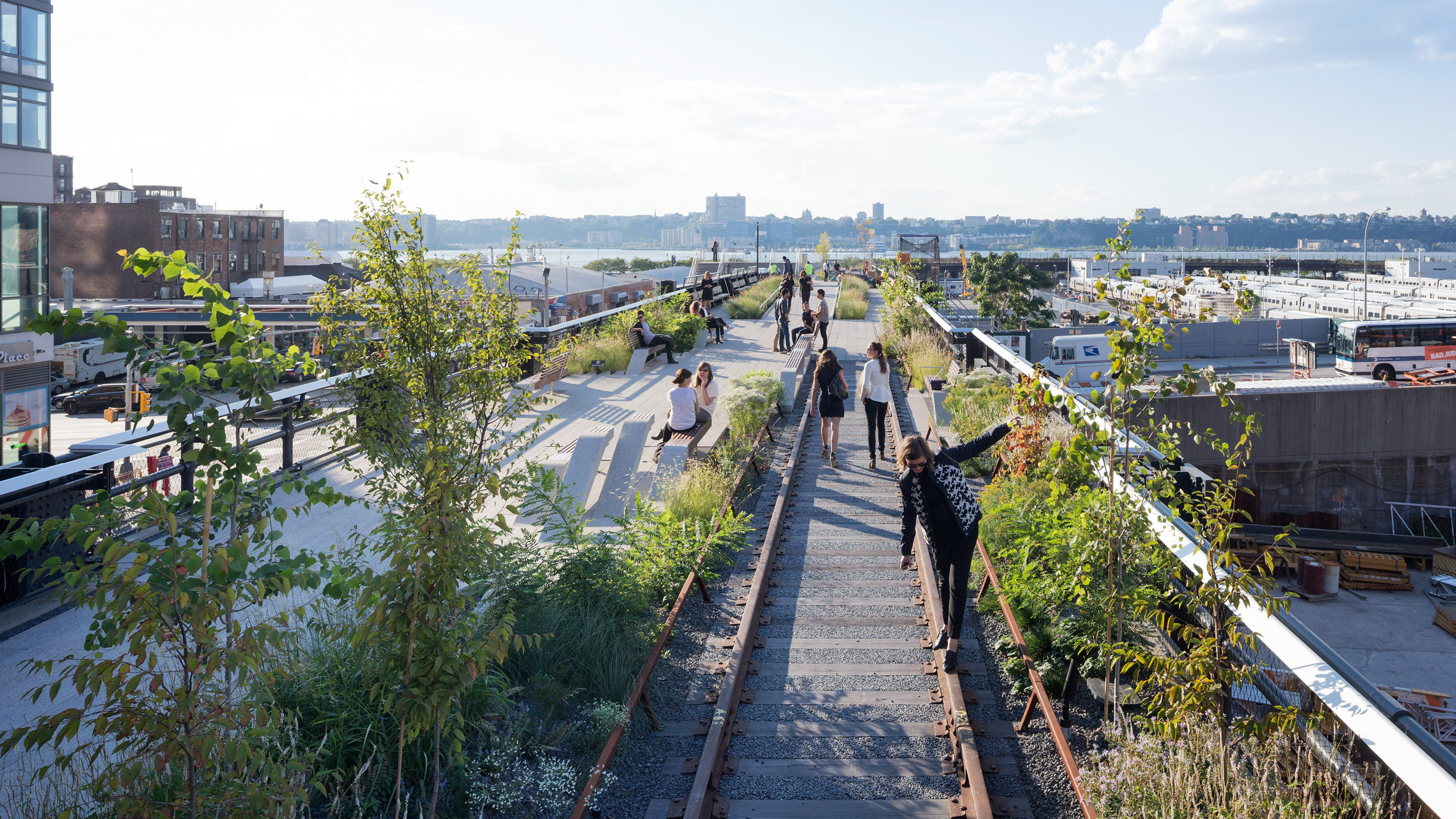The image depicts a vibrant urban scene centered around an old, repurposed railway line that has been transformed into a pedestrian walkway. The railway, now disused and overgrown with foliage and weeds, stretches towards the horizon, flanked by diverse cityscape elements. On either side, businesses and infrastructure—possibly including hospitals, industrial areas, and warehouses—line the scene. Two women and a child are prominently seen walking along the tracks, with the child balancing on one of the rails. Other people are scattered along the path, some sitting on benches and chairs, while others appear to be taking photographs or simply strolling. The right side of the walkway is bordered by a lower level featuring more warehouses, while to the left, the edge of a glass three-story building and a distant brick structure can be seen. An interstate highway, identified by the presence of a mail truck and a bus, runs parallel to this scene, hinting at nearby road activity. The image captures a possible evening setting, indicated by the long shadows and the sun casting its light from the left, illuminating a sky with patches of white clouds and hints of blue. There is also a subtle hint of water in the distance, contributing to the picturesque quality of this urban oasis.